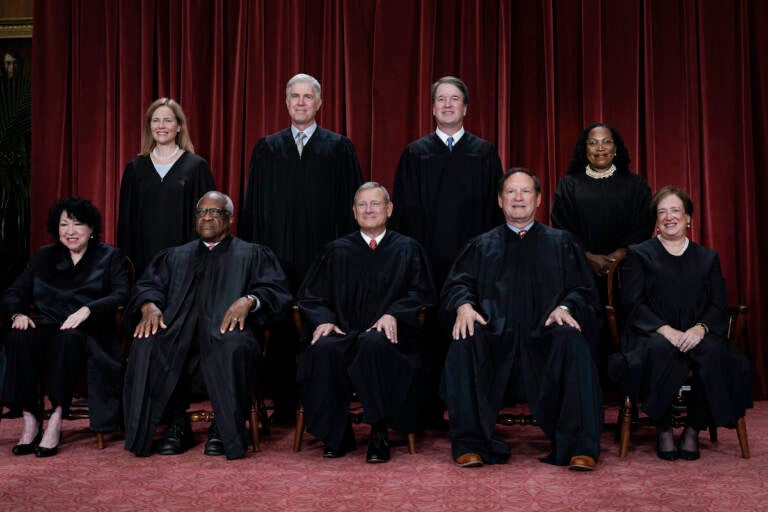This image is an indoor group photo of all nine Supreme Court Justices, arranged in a traditional, professionally lit studio portrait. In the foreground, five justices are seated in wooden chairs, while four justices stand in the background. Behind them, dark red curtains provide a rich backdrop, with a lighter red carpet beneath their feet.

From left to right in the front row: a woman with short black hair, an older man with white hair and black glasses, a man with short gray hair wearing a white shirt with a red tie, a man with short brown hair, and another woman with short brown hair. In the back row, from left to right: a woman with long blonde hair, a man with short silver hair, a man with short dark hair that is graying, and a woman with shoulder-length black hair. All justices are dressed in their traditional black judicial robes.

Notably, most justices appear to be smiling, except for Clarence Thomas, the standing black male on the far left of the back row. The justices are looking at a different angle, suggesting another photographer's presence. The composition and presence of four female justices indicate that this is a recent photo.